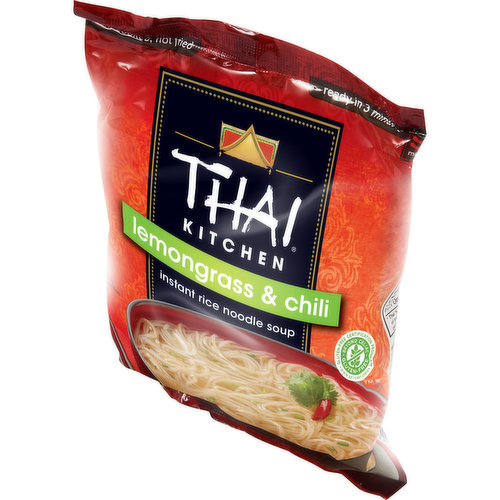The image depicts a package of Thai Kitchen instant rice noodle soup with lemongrass and chili flavor. The package is shown against a white background and is slightly angled, revealing various design elements. The bag is primarily reddish-orange with a patterned background, and features a black square in the center with the brand name "THAI KITCHEN" in large white letters. Below this, there is a green rectangle with the flavor indicated in white letters: "lemongrass and chili." Underneath this, it says "instant rice noodle soup" and displays an image of the noodle soup in a red bowl with a black rim. The top of the package is a tear style and prominently displays "ready in three minutes" in white print. Additional details on the package include a peaked roof-like design above the word "THAI", a black and white decorated border, and a possibly Thai inspection label on the right side, which is green with white and green lettering. The bottom edge of the packaging appears black, and there are white strips and dots as part of the design.